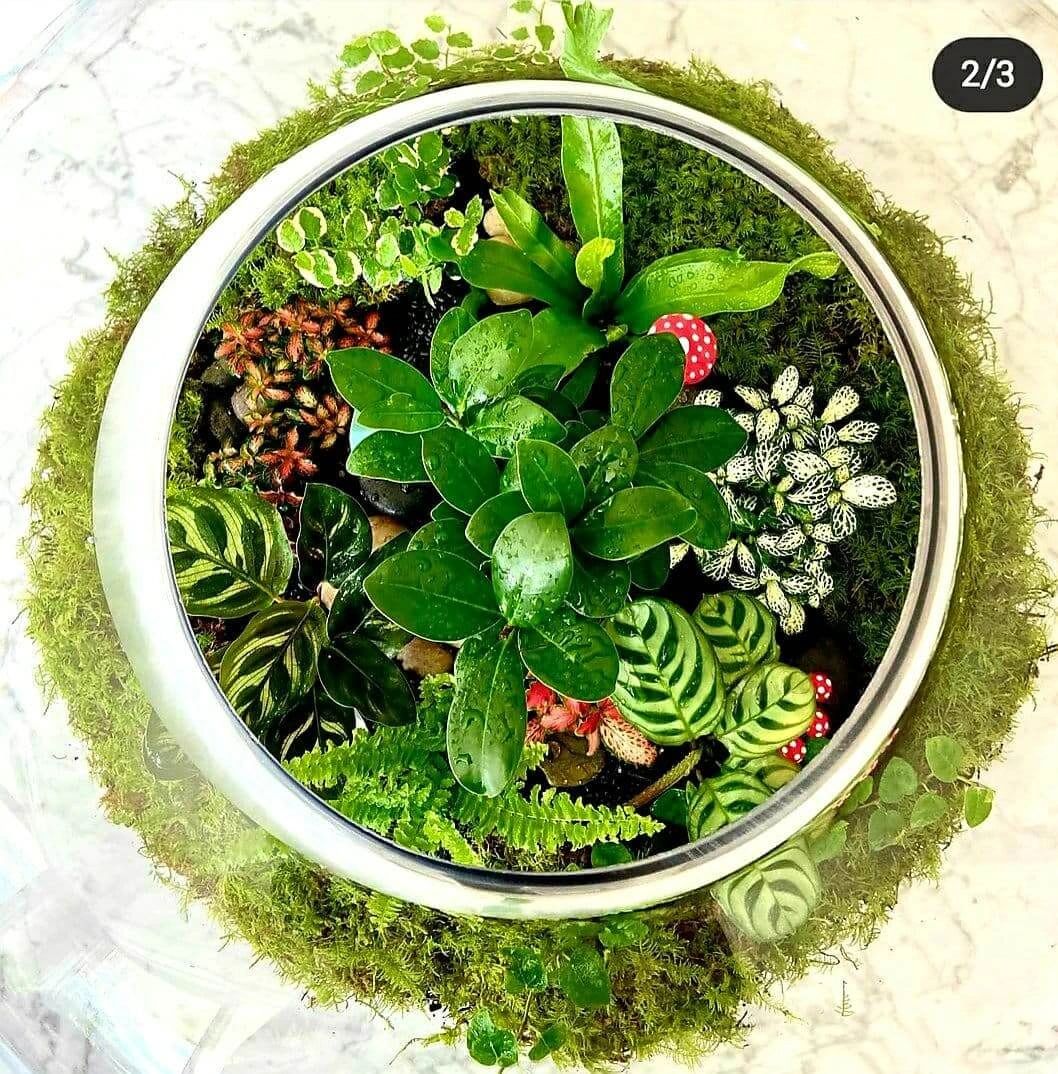This image is a detailed top-down view of an intricately designed planter that gives the impression of a terrarium. The central focus is a variety of green leafy plants, including succulents and ferns, mingled with intricate decorative elements. Among the plants, which range from light green with darker green leaf veining to pale, almost white leaves with black markings, are small, realistic-looking red mushroom caps with white spots. The planter itself, which appears to be white, is surrounded by a base layer of moss and possibly grass. The entire arrangement sits on a white and cream marble or granite countertop. Additionally, there's a notable detail in the top right corner: a small black oval indicating "2/3" in white lettering, suggesting this is the second image in a series of three. The overall scene blends natural and artificial elements, with the plant leaves and decorative mushrooms spilling out to create a visually rich composition.